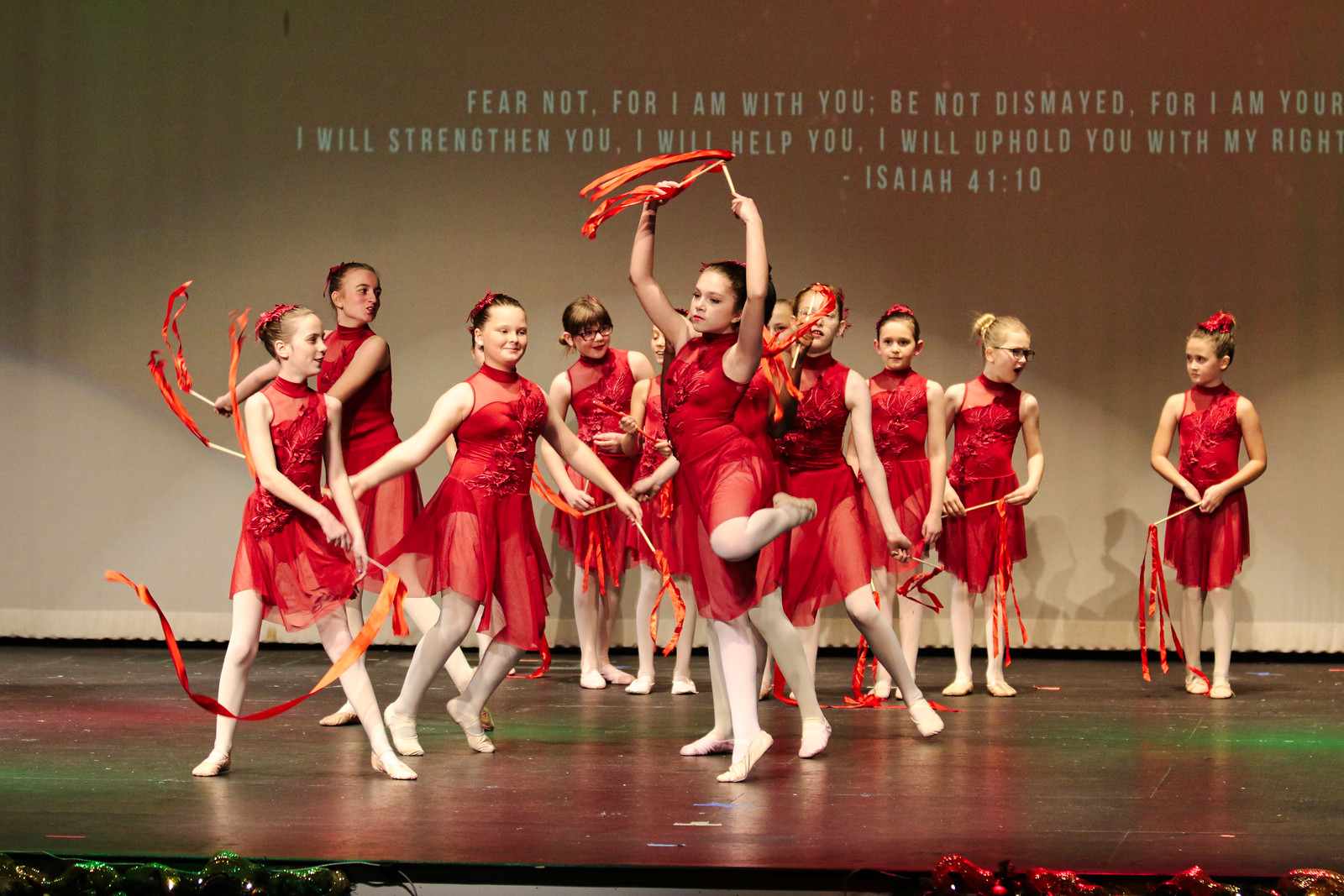The photograph captures a group of young girls, likely between eight to ten years old, performing a dance on a well-lit stage with a black floor. All the girls are dressed uniformly in sheer, sleeveless red dresses paired with white leotards, and their hair is neatly tied back in either high or low buns. They are holding sticks adorned with red or orange ribbons. The performance appears to feature a ballet or dance recital, with the girls arranged facing forward. The center girl is particularly prominent, poised gracefully on her right tiptoe with her left leg bent, holding her ribbon stick above her head. The background features a stage curtain and a partially visible text projection that reads, "Fear not, for I am with you. Be not dismayed, for I am your... I will strengthen you, I will help you, I will uphold you with my right...," which references Isaiah 41:10.